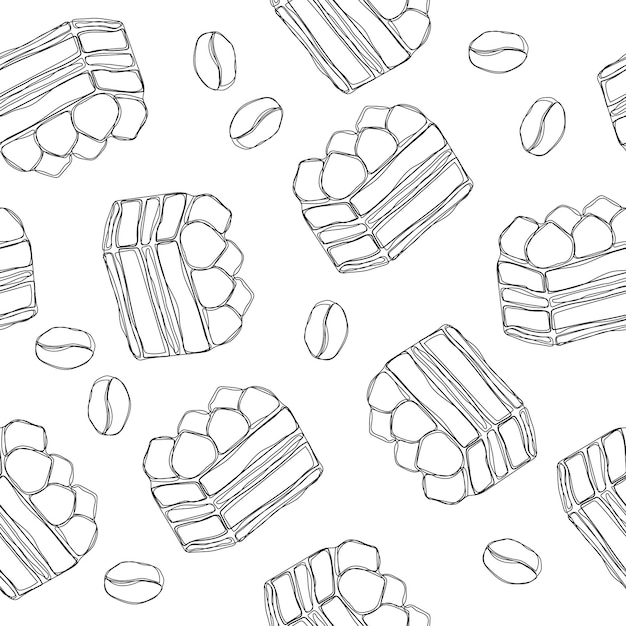In this black-and-white image, we see a detailed drawing featuring multiple rectangular slices of triple-layered cake, adorned with frosting and topped with small, round nut-like decorations. These cakes are scattered and tilted at various angles throughout the scene. Interspersed among the cake slices are numerous coffee beans, also depicted in a similar sketch style. The entire composition of cakes and coffee beans appears to be floating, creating an illusion of them falling through the image. Despite the lack of color, the intricate outlines and consistent design add a dynamic visual rhythm to the picture, with no textual elements present.